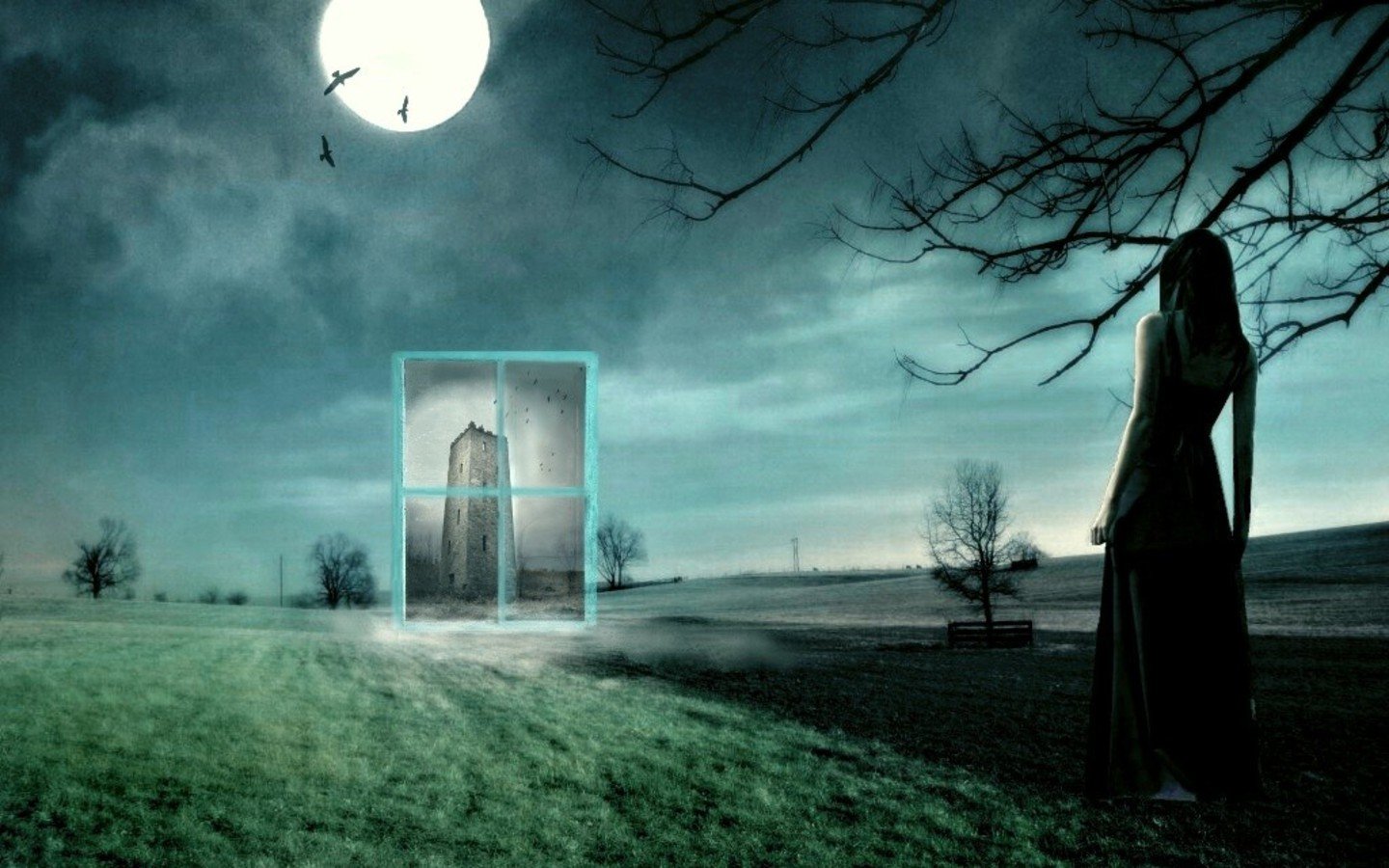In this surreal, composite image, a petite Caucasian woman with long, dark hair stands on the right side, facing away from us, draped in a sleeveless long, dark dress. Her silhouette is shrouded in shadow, with only a faint glimpse of her left arm visible. The background is a dark night sky, transitioning from deep blue to lighter hues where the moon's bright light illuminates the scene. Branches of a tree claw in from the upper right corner, adding to the eerie ambiance. The landscape is stark, with sparse patches of green grass traced by moonlight.

In front of the woman, a mystical window or portal appears, seemingly suspended in space. The frame of this otherworldly opening is teal, featuring a teal cross, and through it, we glimpse a shadowy, gray multi-story building, contrasting sharply with the rest of the scene. Beyond the portal, a full moon sky reveals erratic flocks of birds and bats, enhancing the surreal, almost fantastical atmosphere.